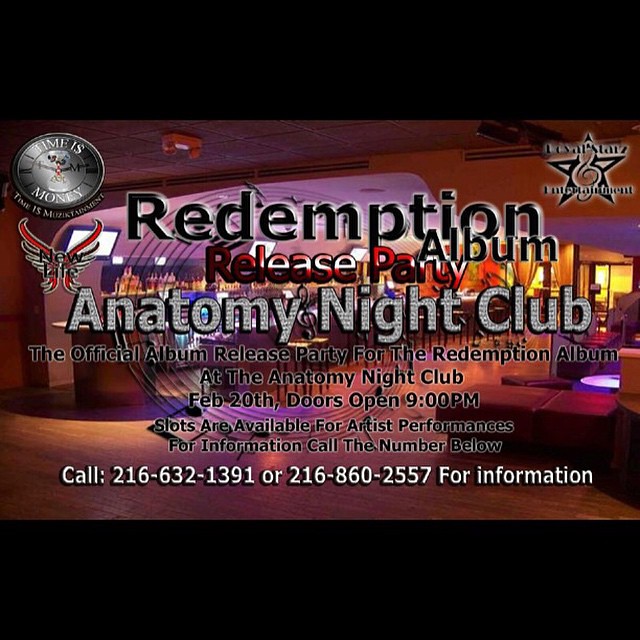This image shows a detailed flyer for the official album release party of "The Redemption Album" at Anatomy Nightclub. The top of the flyer prominently features the text "Redemption Album" in black letters, followed by "Release Party" in striking red letters. At the center, "Anatomy Nightclub" is displayed in clear blue letters. Below this, in black letters, it announces "The Official Album Release Party for The Redemption Album at Anatomy Nightclub, February 20th, doors open 9pm." The flyer mentions that slots are available for artist performances, with the message "For information call the number below" followed by the contact numbers in white letters: "Call 216-632-1391 or 216-860-2557 for information."

The background showcases an image of a nightclub, likely digitally enhanced using Photoshop. Additional design elements include a black star in the upper right corner and a grey clock in the upper left corner with the phrase "Time is Money." The flyer also features ethereal wings and the words "New Life," adding to its dynamic and vibrant aesthetic.